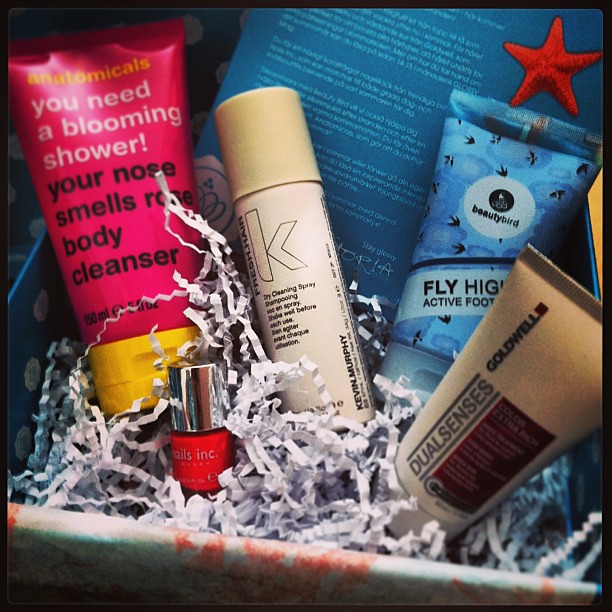This square photograph captures the interior of a gift package filled with various skincare products, nestled inside a blue box adorned with white polka dots. The box is padded with delicate, accordion-folded white confetti, which creates an elegant and protective cushion for the items. Toward the left, a bright pink bottle with a yellow cap prominently displays the label "Anatomicals: You Need A Blooming Shower, Your Nose Smells Rose, Body Cleanser." Just below it sits a small orange bottle of nail polish with a shiny silver cap. To the right, there is a tan, cylindrical tube marked with the letter "K," followed by another tube labelled “Dual Senses.” Additionally, a narrow blue spray bottle is visible, and in the bottom right corner, a tan bottle completes the assortment. The background features a large blue note, though the text on it is too blurry to decipher. Above these items, a red star accents the arrangement, adding a festive touch. The contents are beautifully arranged, making the package a delightful visual treat.